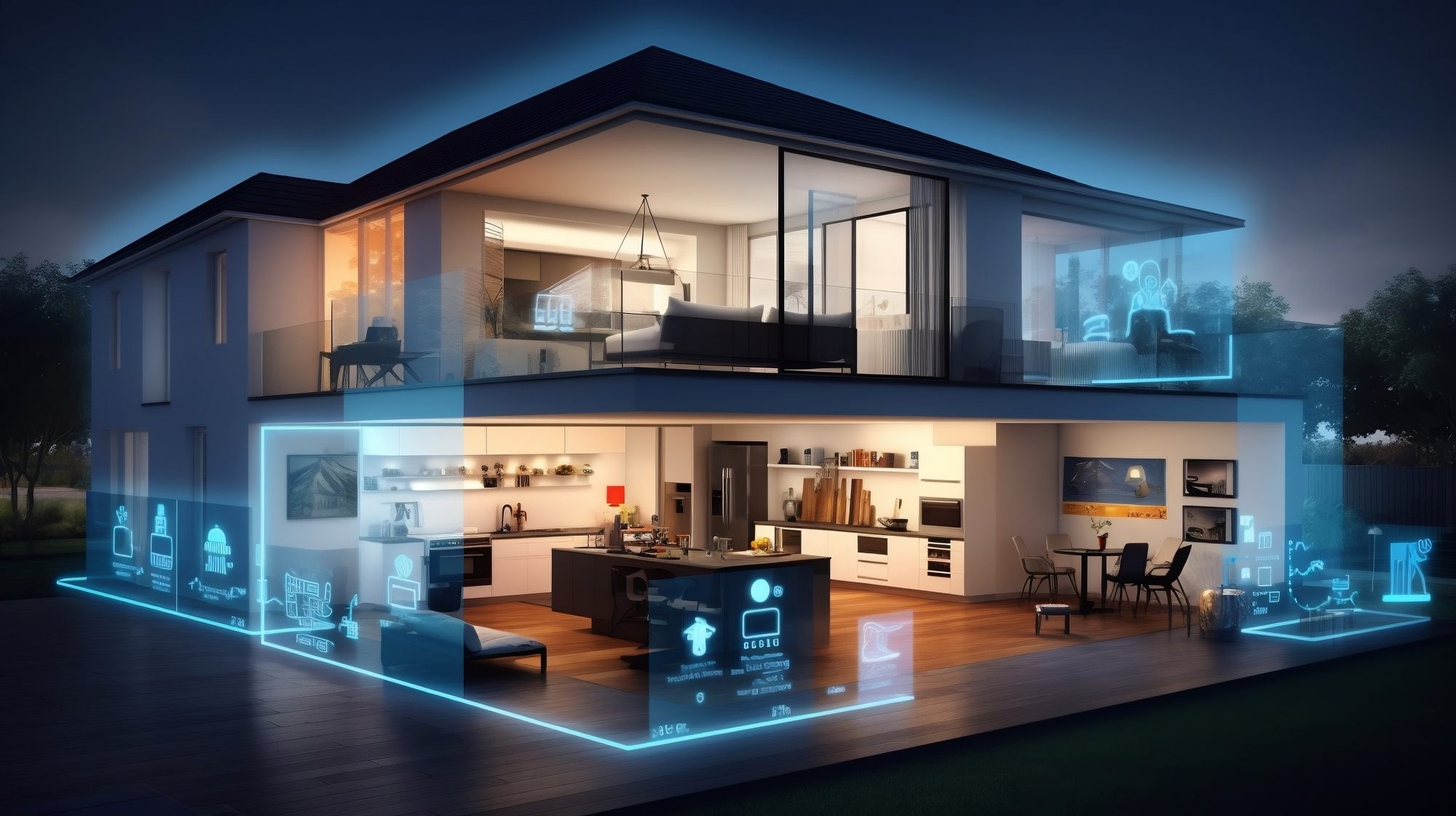The image depicts a stunningly futuristic and ultra-modern double-story building, possibly a digital graphic or game environment. The architecture features exceptionally clean and sparse lines, accentuated by blue LED lights outlining the structure and holographic images superimposed around the edges. The building's entire front facade, likely of a business or residential nature, is made of glass, allowing an unobstructed view inside. On the ground floor, one can see a vast, open space that resembles a kitchen area, complete with an island, refrigerator, stove, sink, counters, and a small circular dining table with four chairs. The second story, also glass-fronted, reveals what appears to be a master bedroom, furnished with a large bed facing the back and a balcony. The setting is against a stark black night sky, with trees flanking the sides of the house and a wooden platform extending both inside and outside. The scene exudes a blend of futuristic technology and minimalistic design, lending it an ambiance that could easily be part of a game.